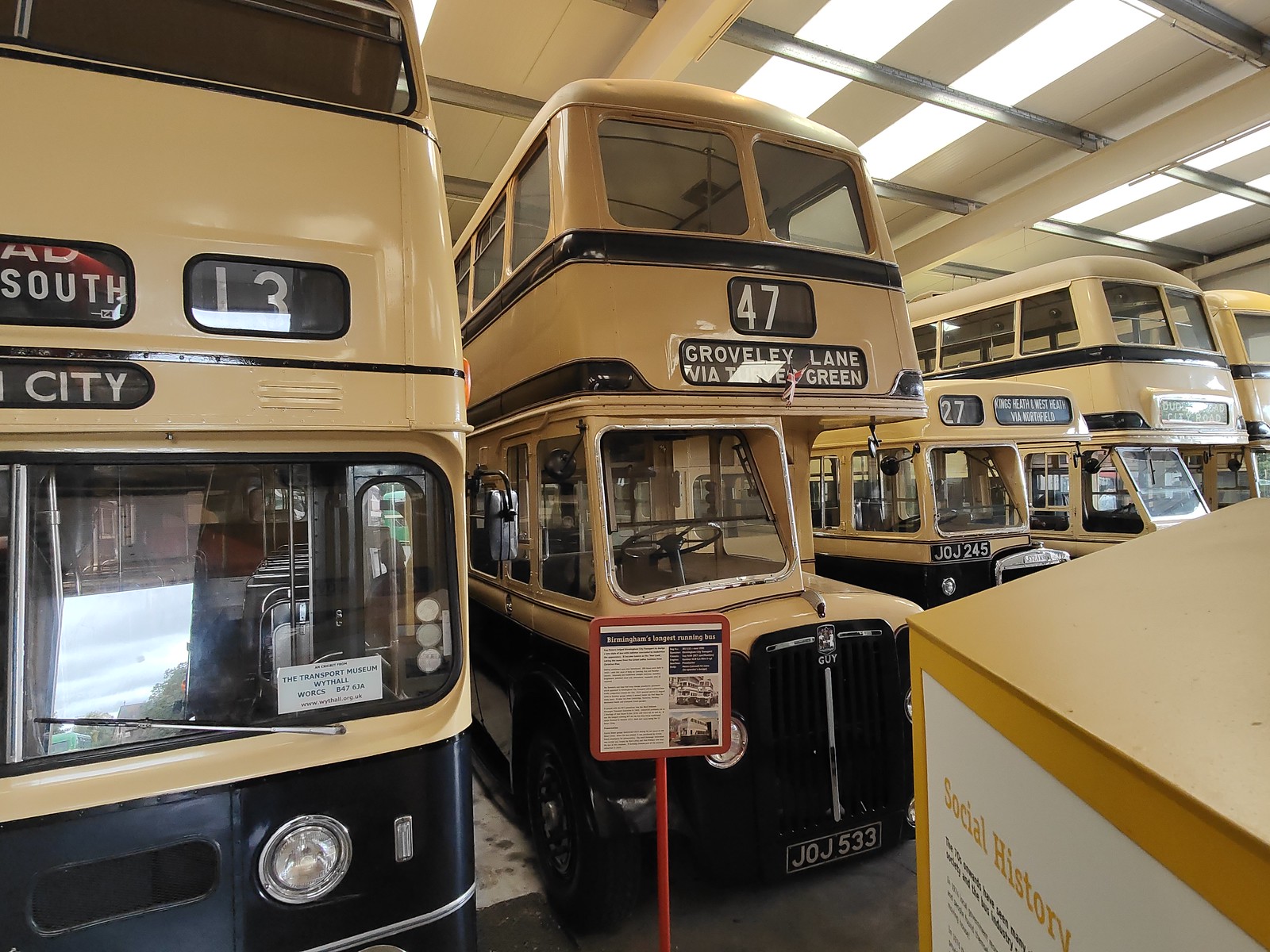This image is a detailed view of five buses displayed from the front in what appears to be a museum setting. The buses are parked and unoccupied, showcasing their historical designs. Four of the buses are double-decker style, featuring a beige upper deck and a black lower deck, while one single-decker bus is positioned among them. 

On the far left, a double-decker bus displays a destination sign reading "South City" and is numbered 13. Immediately to its right, another double-decker bus indicates it is heading to "47 Grovely Lane." In the center, the single-decker bus, painted in the same beige and black color scheme, bears the number 27. Further to the right, two additional double-decker buses can be seen in the background. 

In the bottom right corner of the image, part of a sign is visible. It has a white background with text in yellow, reading "social history." The setup suggests a historical exhibit focusing on the evolution and significance of public transportation.